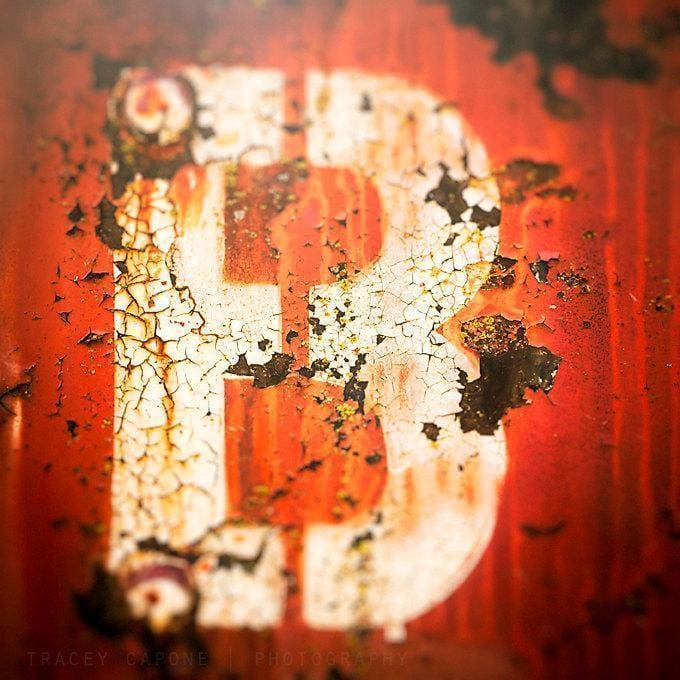This photograph is a close-up of a weathered and dilapidated sign, prominently featuring a large, white-painted letter "B" at its center. The red background of the sign is extensively corroded and rusted, especially concentrated in the upper right corner and the area immediately to the right of the letter. The letter "B," though originally white, shows significant signs of age, with yellowing, rust-colored discoloration, and a distinctive web-like crack running down the middle. The crack has caused parts of the letter to chip away, leaving the red background exposed in places and giving the impression that the image has been poorly maintained over time.